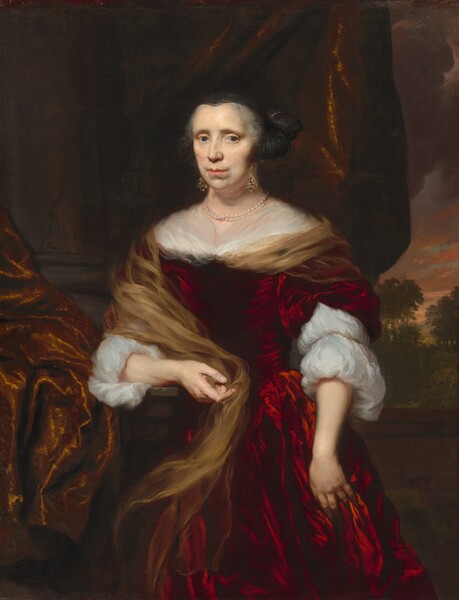The painting is a classical-style portrait of an elderly white woman, evoking the Renaissance era, possibly displayed in a gallery or museum. The woman has a complexion of very fair white skin, with dark eyes and pink lips. Her expression is one of dignified neutrality, suggesting she was perhaps caught off guard during the sitting. She wears a luxurious dark red velvet dress adorned with white lace around her shoulders and biceps, and a see-through white wrap draped over her shoulders. A pearl necklace adorns her neck.

Her hair appears to be up but is intriguingly intertwined with a brownish-gold sheer scarf that flows from her chest, over her right shoulder, around her back, and cascades down her left side to just below her knees. Her right hand hangs straight down while her left hand is bent near her stomach with slightly open fingers.

The background is predominantly dark, contributing to the painting’s oblique atmosphere. To the right, the dim scene reveals distant trees under a sky painted in orange and yellow hues, reminiscent of a sunset. On the left, a dark drape or curtain, possibly in shades of dark brown to amber, adds to the rich, somber ambiance of the setting.